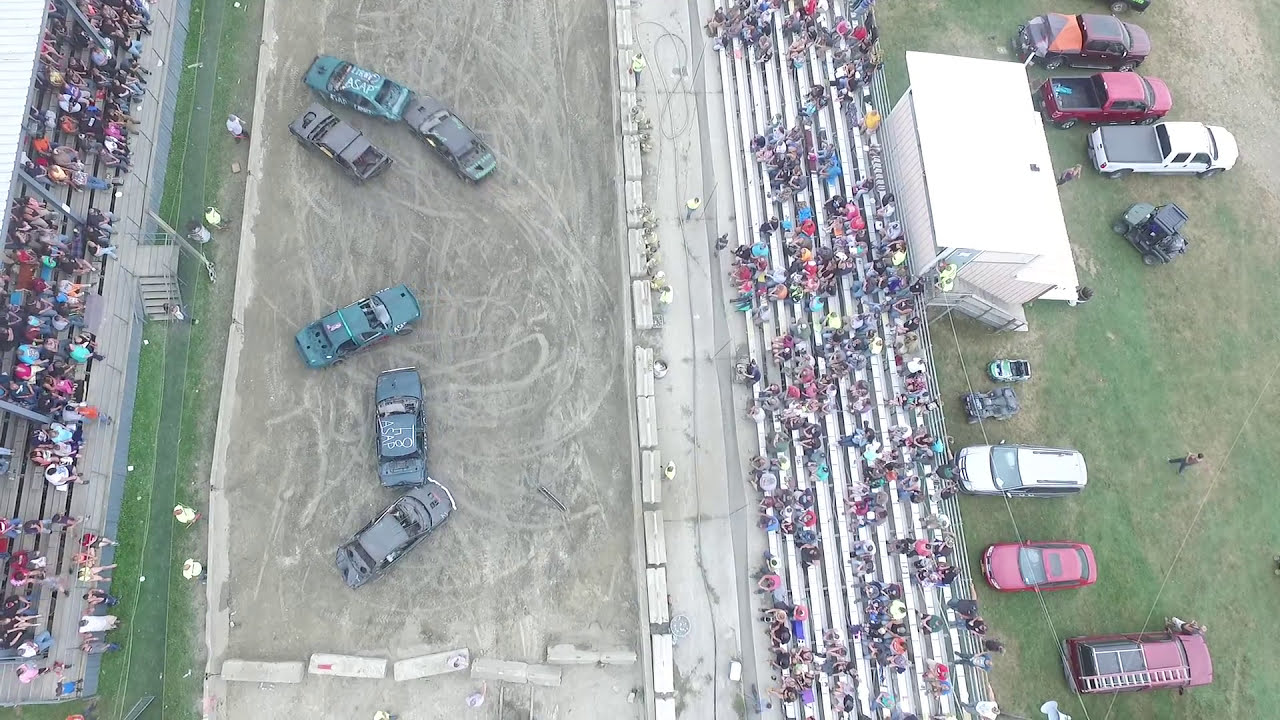This aerial photograph, taken outside on a cloudy day, provides a detailed view of a lively demolition derby event. The scene is dominated by a large, light brown dirt area that spans vertically from the bottom to the top of the image, situated on the left side. In the center of this rectangular dirt lot, six old, battered cars in dark green and black—some marked with white graffiti and lacking windshields and windows—are positioned. A myriad of tire tracks crisscross the ground, hinting at the chaotic nature of the event.

Flanking this dirt arena, there are bleachers on both the left and right sides filled with dozens of spectators, many of whom are clad in bright colors. The left bleachers appear to be made of light gray metal or concrete, while the right bleachers are smaller and white. Beyond the right-side bleachers, a white building with a white roof is visible near the top right corner of the image.

Behind these bleachers, a patched grassy area featuring both green grass and brown dirt can be seen, peppered with several parked vehicles, including red and white cars as well as ATVs. People are walking around this peripheral area, adding to the vibrant activity and energy of the scene. The overall context and specific details suggest the image captures a demolition derby, a popular event often associated with the southern United States, emphasizing the designed-for-destruction cars and the dynamic, bustling atmosphere.